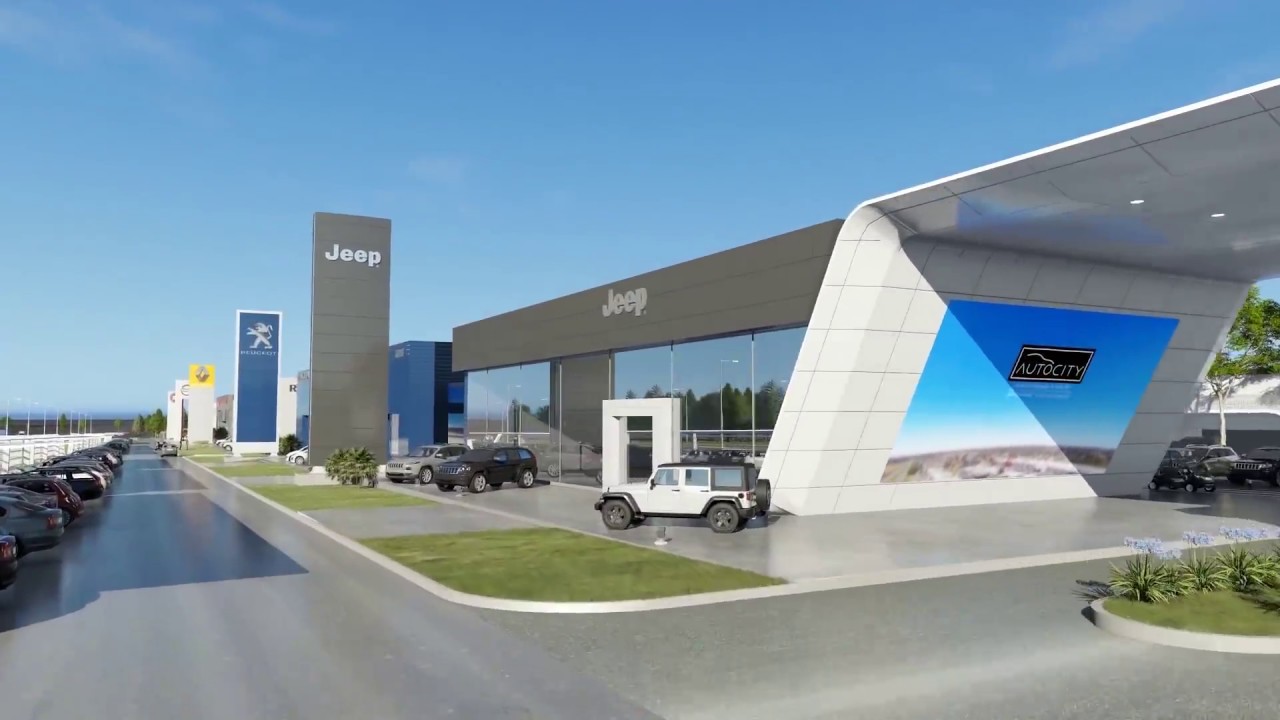The image is an outdoor professional shot of a modern Jeep dealership, prominently displaying its well-maintained front entryway. The dealership building, in gray and white tones, features large open glass windows through which displayed vehicles for sale can be seen. A large digital screen sits under a stylish white overhang, enhancing the dealership's modern aesthetic. The meticulously landscaped grounds boast colorful flowers, mowed green grass, and a clean parking lot with neatly lined-up cars in various shades, including white, dark gray, and light gray. Large, clearly visible Jeep signs and symbols are scattered throughout the area. The sky is bright and clear blue, highlighting the sunny day and contributing to the fresh, inviting atmosphere of the dealership. The photo, taken from an angled perspective, captures the essence of the dealership’s outdoor environment, blending vehicular display, aesthetic architecture, and pristine landscaping seamlessly.